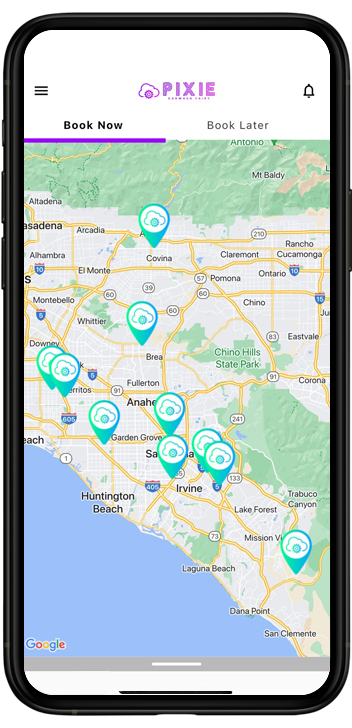The image showcases a smartphone displaying a detailed map via a mapping application titled "Pixie." The map depicts the coastal region of California, focusing on the eastern coastline. Key cities and highways, highlighted with yellow lines, are prominently featured alongside green landmasses and the blue expanse representing the ocean.

Beneath the map, there is a white rectangular banner containing three distinct options for various locations. Each option includes a thumbnail with three images related to the respective place. The first location, "Five Star Mobile Detailing," appears on the left. The middle option showcases "Magic Brush Car Wash," while the third option on the right lists "Garage G.H.A." This detailed view offers users a comprehensive look at the geographic layout and potential service locations along California's coastline.